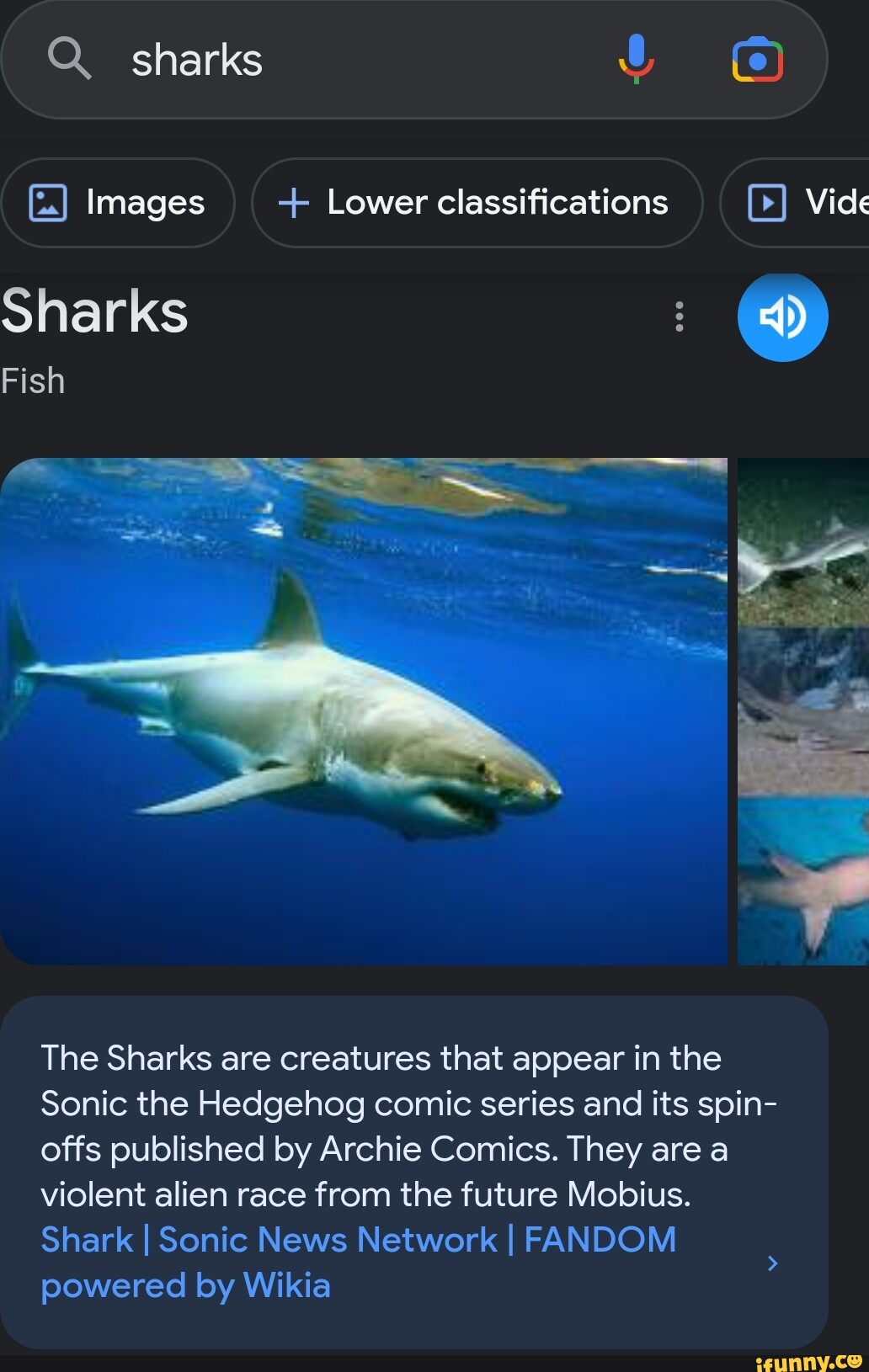The image is a screenshot of a search query for sharks. At the very top, in a dark gray oval, there is a magnifying glass icon on the left side. To the right of the magnifying glass, the word "sharks" is displayed, followed by a microphone icon and a Google Lens icon. Below this, three categories are listed: Images, Lower Classifications, and Videos. Only part of the word 'Videos' is visible, showing the letters "V-I-D-O."

Directly underneath, the term "sharks" is highlighted, and the word "fish" is displayed next to it. To the right of "fish" is a blue circle containing a speaker icon. To the left of the speaker icon are three small gray vertical dots.

Below this section, an image of a shark swimming in dark blue water is visible. The shark is light gray and shown from a side view. Next to this image is a partial image, with only about 10-20% of it visible on the right.

Further down, white text states: "The sharks are creatures that appear in the Sonic the Hedgehog comic series and its spinoffs published by Archie Comics. They are a violent alien race from the future, Mobius." Beneath this text, a blue-gray rectangle contains blue text reading: "shark / Sonic News Network / fandom powered by Wikia." In the bottom right corner of the image, the text "ifunny.co" is displayed in yellow.